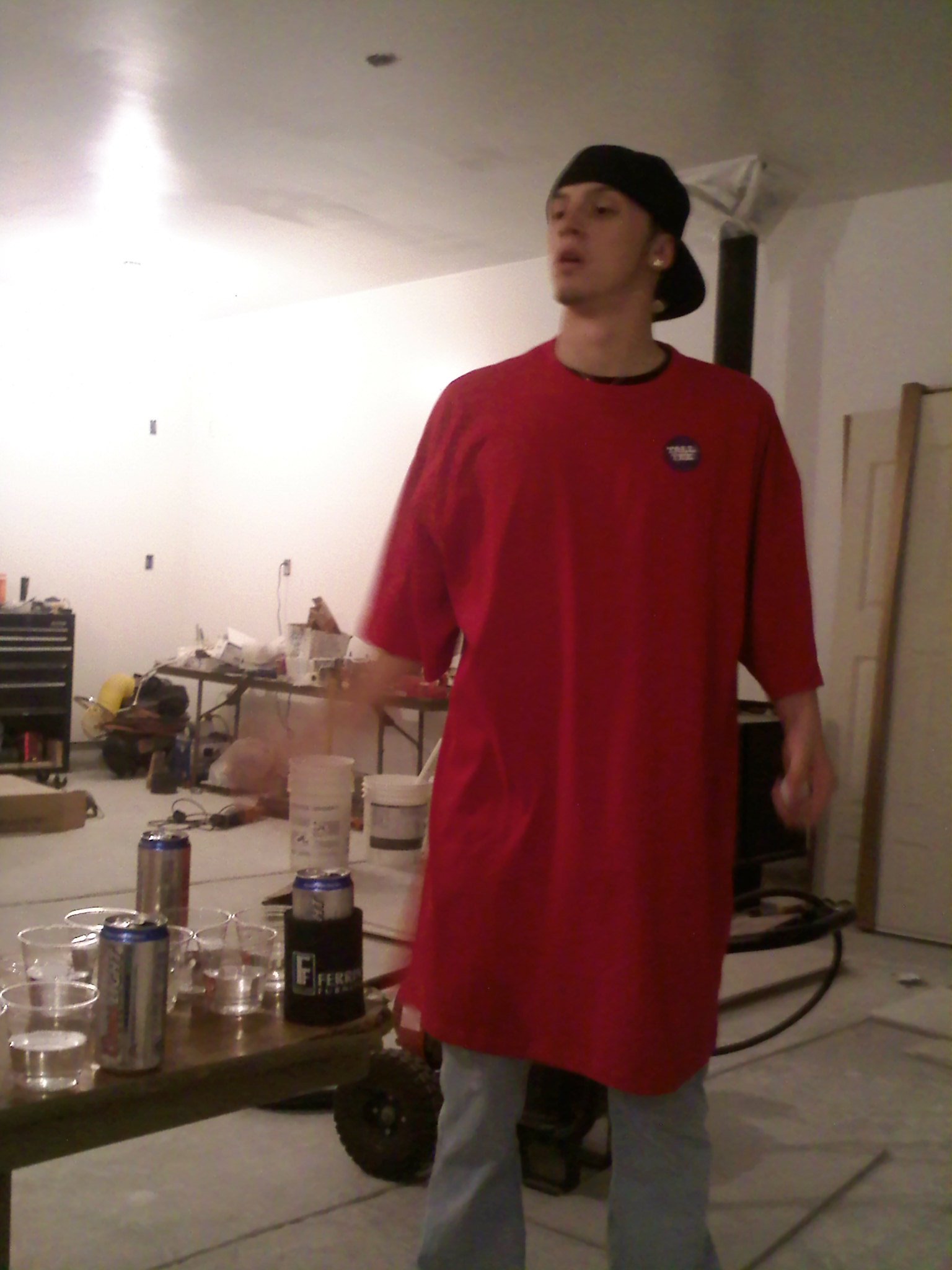In a cluttered, unfinished basement with white walls and a white ceiling, a young man is standing under a bright spotlight mounted on the top left corner of the room. He is wearing an oversized, knee-length red t-shirt with a logo on the left chest, its short sleeves extending below his elbows. He also sports light wash blue jeans and a black baseball cap worn backwards, with a sparkling diamond earring adorning his left ear. His facial hair includes grown-out sideburns and a light goatee, accentuating his thin frame. The man looks towards the bottom left, his mouth slightly open as if in mid-argument, giving off a tense, confrontational vibe. Behind him, the room appears messy and disorganized, with two tables cluttered with household items, including open Coors Light beer cans, plastic glasses filled with clear liquid, and various boxes. A black garage cabinet and a closed toolbox lean against the far wall, suggesting the space might double as a makeshift party area and workspace.